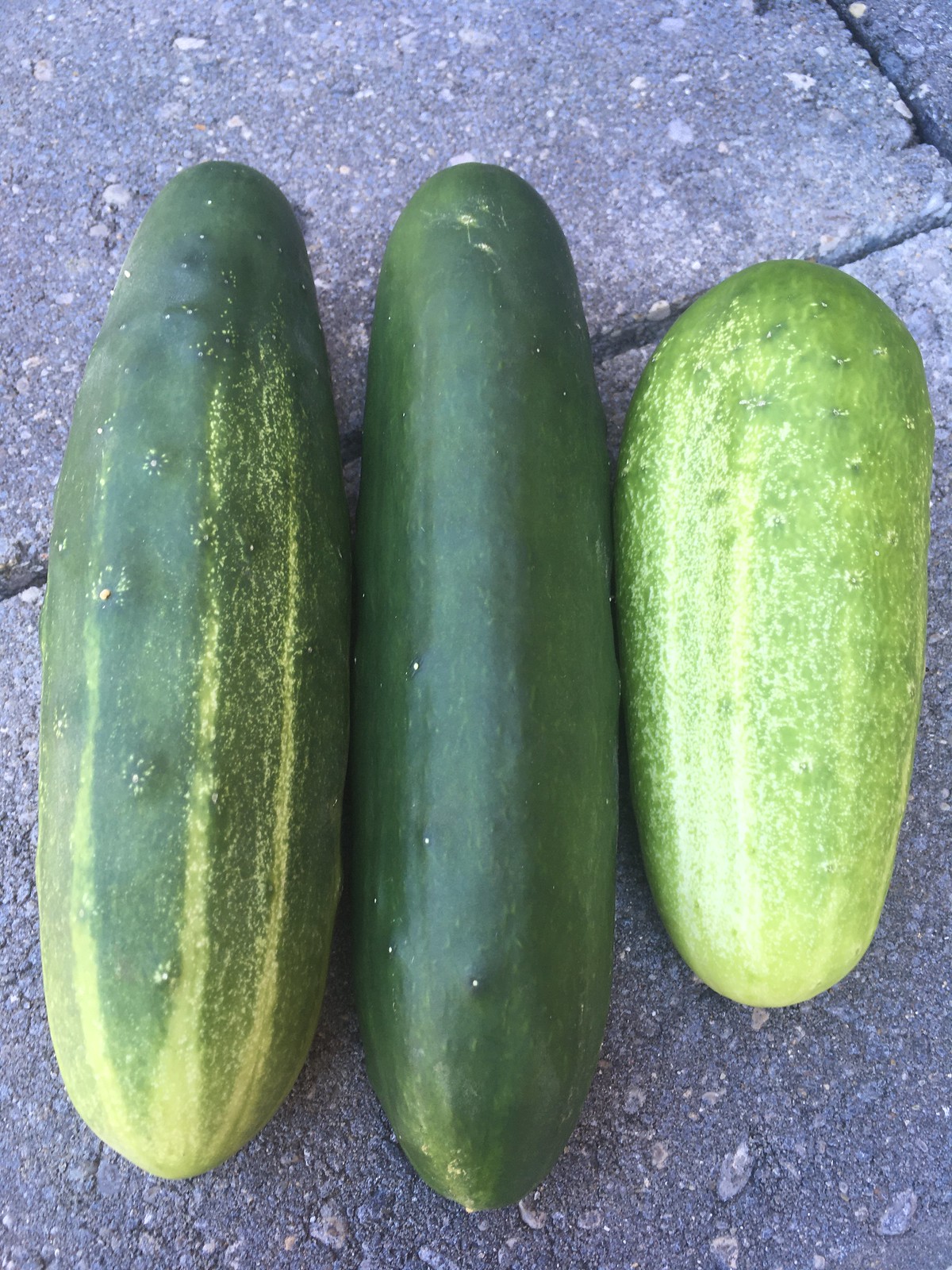The photograph captures three cucumbers lying side by side on a dark gray stone pavement speckled with lighter gray and brown. The middle cucumber is the longest, characterized by a mostly dark green color with specks of light green at its top and bottom. The cucumber on the left is slightly shorter, medium green with yellowish-light green stripes, and has raised bumps scattered across its surface. The cucumber on the right stands out with its stunted, short, and round shape, sporting a light green color interspersed with white streaks and a speckled appearance. The pavement beneath them reveals cracks between individual bricks, adding texture to the image, which was taken during daylight. The cucumbers appear dry and ripe.